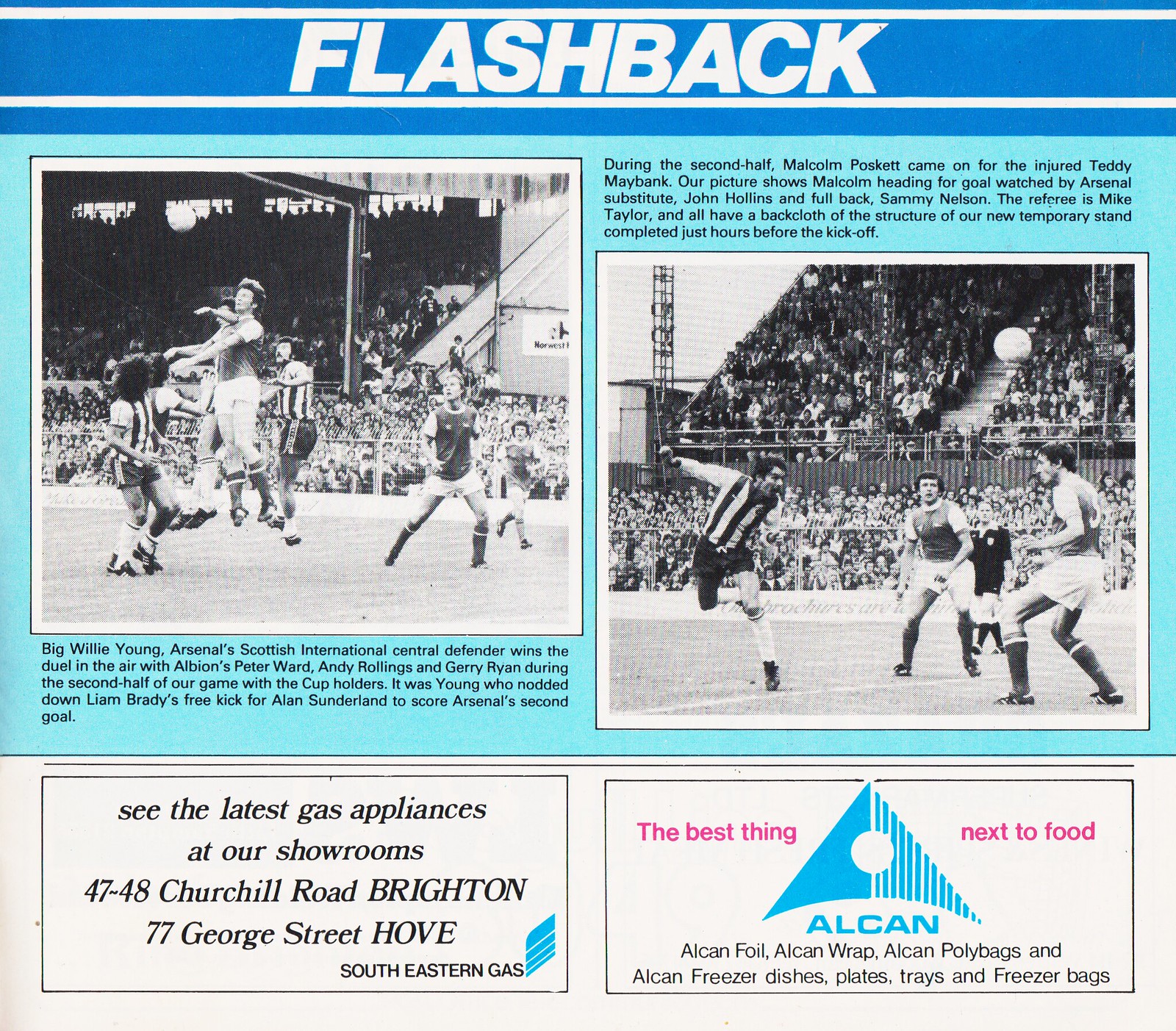This image appears to be a vintage page from an English football club's official program. At the top, it prominently features the title "Flashback" in white text against a blue strip.

The page showcases two black and white photographs. The left photo depicts Big Willie Young, Arsenal's Scottish International central defender, leaping into the air among a cluster of players including Pete Ward, Andy Rollins, and Jury Ryan, all of whom are competing to head a football. The caption notes that Young won this aerial duel during the second half of their match against the cup holders and set up Arsenal's second goal by nodding down Liam Brady’s free kick for Alan Sunderland.

The right-hand image captures Malcolm Poskitt mid-strike, with the ball soaring high above the other players. This scene occurred during the second half after Poskitt subbed in for the injured Teddy Maybank. The caption mentions that the photo shows Poskitt heading for the goal, observed by Arsenal substitute John Hollins and fullback Sammy Nelson, with referee Mike Taylor also in the frame against the backdrop of a newly completed temporary stand.

At the bottom of the page, there are two advertisements. The left advert promotes gas appliances, available at a showroom located at 47-48 Churchill Road, Brighton, and 77 George Street. The right advert highlights Elk and Ekol products, including foil, wrap, poly bags, freezer dishes, plates, trays, and freezer bags.